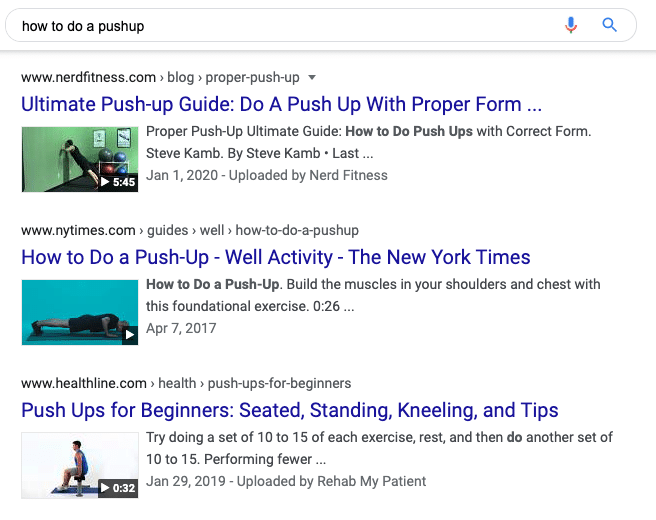A detailed screenshot displays a Google search for "how to do a push-up" on a digital device. The Google search bar is prominently featured at the top, complete with a microphone icon on the right and a magnifying glass icon to the right of it. Inside the search bar, the query "how to do a push-up" is typed in black lettering.

Below the search bar, three search result entries are visible:

1. The first result features a thumbnail of a video showing a man in black shorts and a tank top leaning against a green wall, with medicine balls in the background. Overlaid on the thumbnail is the title "Ultimate Push-up Guide: Do a Push-up with Proper Form" in blue text. To the right of the thumbnail, the description reads "Proper Push-Up Ultimate Guide: How to Do Push-Ups with Correct Form" by Steve Cam. The description ends with an ellipsis and the date "January 1st, 2020." This entry was uploaded by Nerd Fitness.

2. The second result presents a thumbnail of a man dressed in black attire—shorts, shoes, and a shirt—lying on what appears to be a yoga mat, preparing to do a push-up. The title "How to Do a Push-Up: Well Activity" is highlighted in blue. Below the thumbnail, the description states, "Build the muscles in your shoulders and chest with this foundation exercise." The date for this entry is listed as "April 7th, 2017," and it was published by The New York Times.

3. The third result's thumbnail shows a man in a blue tank top and gray shorts sitting on a workout bench, with a blue mat under his feet. He is wearing white sneakers. The title "Push-Ups for Beginners: Seated, Standing, Kneeling, and Tips" is displayed in blue. To the right, the description encourages, "Try doing a set of 10 to 15 of each exercise, rest, and then do another set of 10 to 15." The description trails off with an ellipsis, and the date "January 29th, 2019," noting that this content was uploaded by Rehab My Patient.